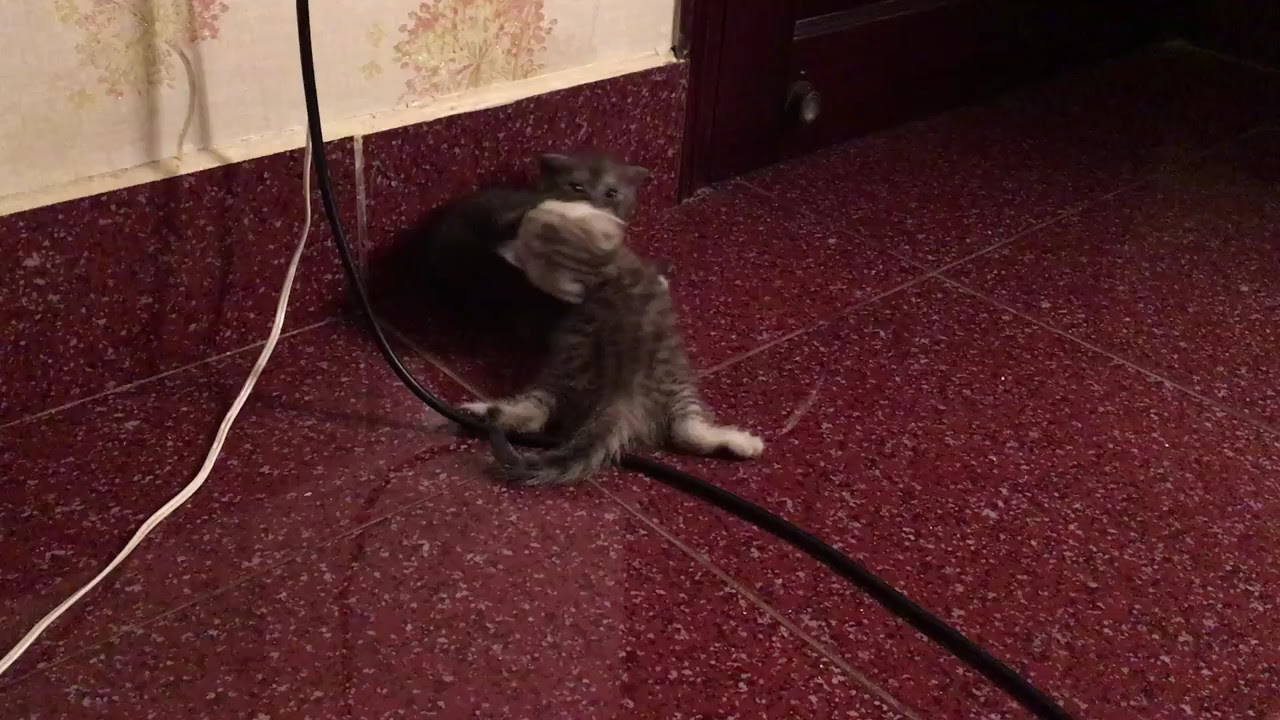In this image, we see two playful kittens in the center of a room with textured red tile flooring. The tiles are a vibrant cherry red adorned with white and black sparkles, enhancing their texture. One kitten is solid black and positioned in the background, with its eyes and ears peeking out, while the other kitten, primarily gray with stripes and white patches, is in the foreground, intertwining with the black kitten. The grey and white kitten's back legs and tail are distinctly visible. A black and white wire is running partially across the floor from the top left, adding to the indoor setting, which seems to be inside a house, possibly a living room. The room also features a maroon baseboard matching the tile and cream-colored wallpaper above it. In the top right, there's a doorway indicating another room. The overall scene captures the innocence and energy of the kittens as they engage in playful antics on the colorful, textured flooring.